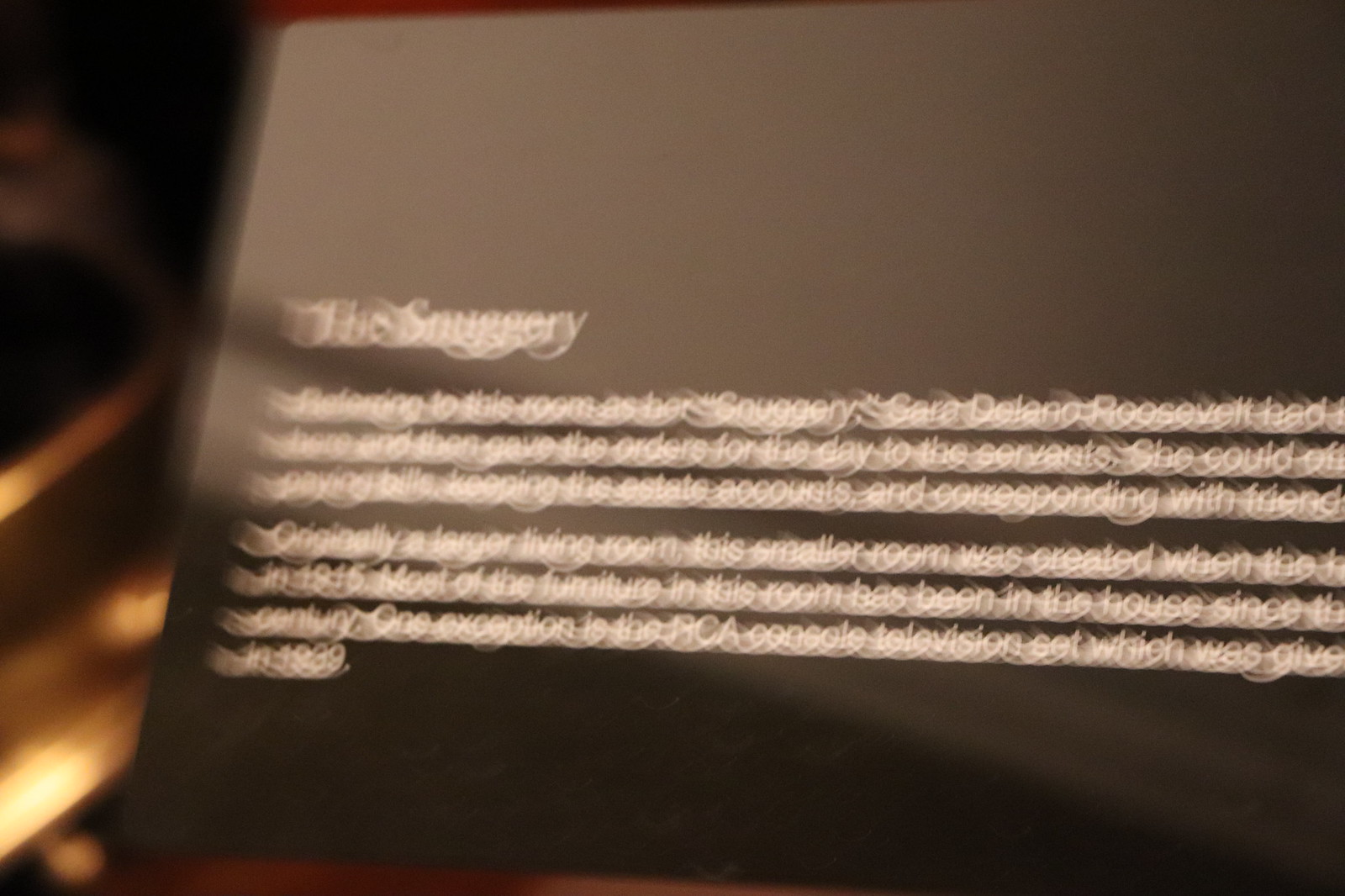This horizontally-oriented rectangular image depicts a blurry and blackened photograph, reminiscent of a double vision effect. The focus is a black plaque, illuminated subtly by lights in front of it, though the lights themselves are not visible in the image. The text on the plaque is mostly indistinct due to the blur, but a few words can be deciphered. The prominent word appears to be "Saugery," spelled as S-O-U-G-G-E-R-Y. Below that, in much smaller print, the name "Sarah Delano Roosevelt" is partially readable on the first line. On the second line, the centered word "servants" can be distinguished, as can the phrase "she could." Further down, the term "friend" is legible. Additionally, the text "originally a larger living room" stands out. This smaller room was created when the], and most of the furniture in this room has been in the house since] can be partially read. The final visible phrase notes one exception being a console television set that was given. The overall impression of the image is one of obscured historical information and a sense of antiquity, conveyed through the indistinct text and dark tones.